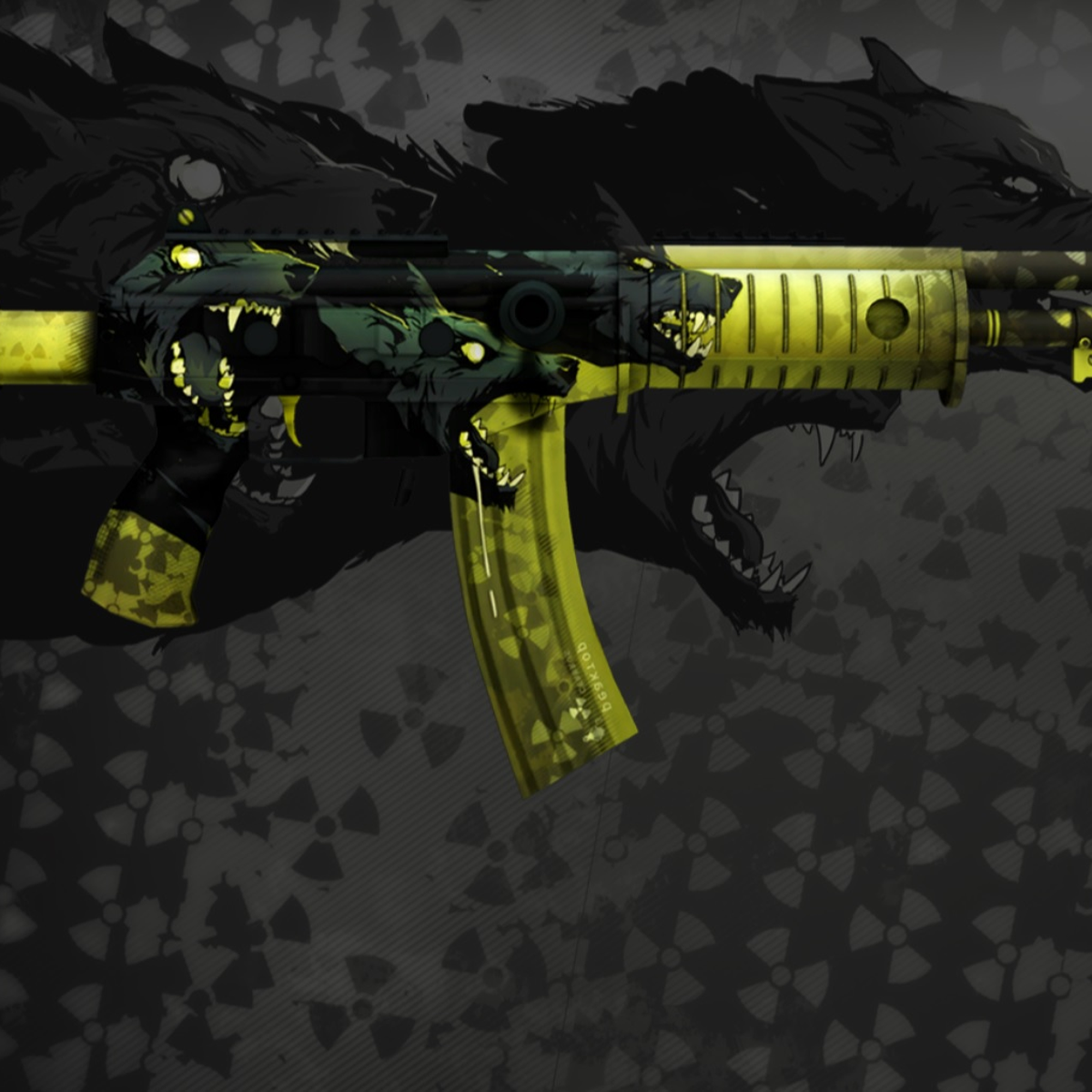This image appears to be of an assault rifle, but it is stylized, giving the impression it could be a skin for a video game like Fortnite or Call of Duty. The rifle features distinctive artwork with three snarling wolves. The wolves, depicted in both the background and on the rifle, have greenish teeth, eyes, and patches of fur, while the rest of their bodies are black and gray. The gun itself has various yellow elements – including parts of the pistol grip, the magazine, the stock, and the hand grip under the barrel – which are marked with the nuclear radiation symbol. The background is a chaotic mix of gray and black splotches, echoing the fierce energy of the wolves. The entire aesthetic combines a sense of danger with a vivid color scheme, making the rifle stand out as both a menacing and visually striking piece.